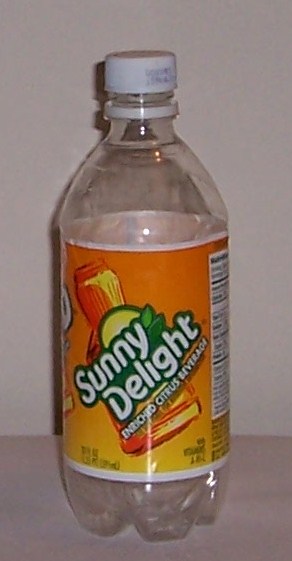The image features an empty clear plastic bottle of Sunny Delight Enriched Citrus Beverage. The bottle is positioned on an off-white or gray surface with a white or beige background. The front of the bottle prominently displays an orange and yellow label with "Sunny Delight" written diagonally from the bottom left to the top right, outlined in green. Below "Sunny Delight," it reads "Enriched Citrus Beverage" in smaller white print. A white cap seals the top of the bottle. To the right side of the label, part of the nutritional information is visible, and on the left edge, a fragment of a white circular letter, likely part of the repeated branding from the reverse side, can be seen. The label also features an image of a sun behind the text that fades from orange to yellow near the bottom.